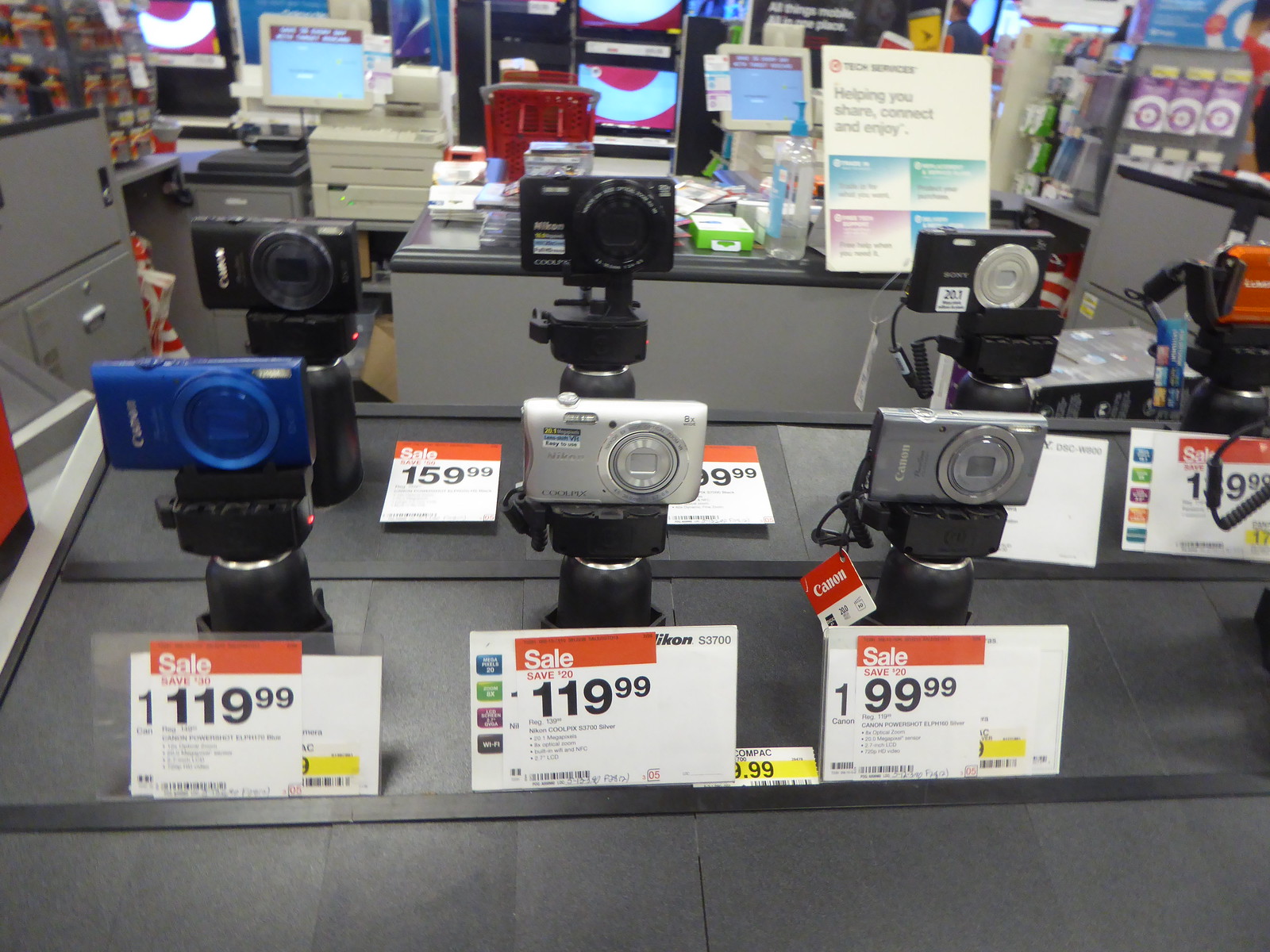This is a digital photograph taken inside a Target store, specifically in the electronics department. The image prominently features a display of small, rectangular digital cameras set on a gray countertop that has a slightly darker gray border. Each camera is placed on a black plastic stand and features a sales tag in front of it. The tags have a red border with "SALE" written in bold white letters, and the price listed underneath in black print. 

On the display's bottom row, there are three cameras: a dark blue camera on the left, a silver camera in the middle, and a darker silver one on the right, with respective sale prices of $99.99, $119.99, and $159.99. The top row features three black cameras, one of which has a silver front panel. On this row, there's also an orange camera. In addition to these, there are further electronics and products visible in the background, including TVs and various store fixtures. You can see two cash registers with white, black, and gray hues, underscoring the retail setting.